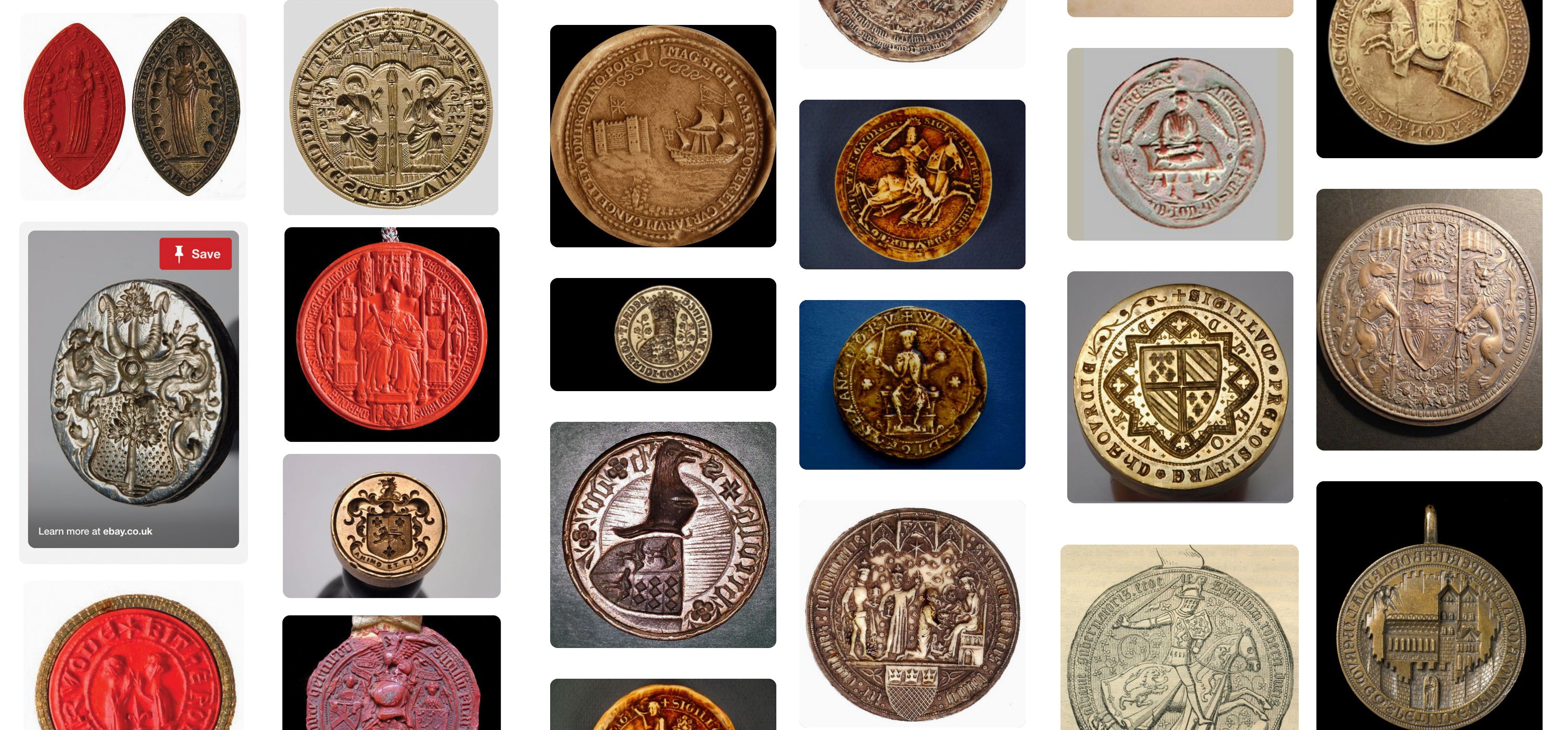This overhead collage features a meticulously arranged collection of various historic and cultural medallions and coins. Organized into six rows, the assortment showcases a variety of items, primarily circular in shape, though a few are football-shaped. The first row contains three items, including two football-shaped medallions at the top—one red and one gold—followed by a silver circular coin beneath them, and a red coin further down. Moving to the second row, there are four coins in gold, red, white, and purple hues.

In the third row, from top to bottom, there is a gold coin, a silver coin, a white coin, and the top section of another gold coin. The fourth row's highlights include the bottom of an old rusted coin, a gold coin featuring a horse and a rider, and a gold coin depicting a man sitting in a chair, holding a stick and a ball, followed by a silver coin with multiple figures on it.

The fifth row begins with a silver coin showing a seated man at a table. The second coin is gold, resembling a ring with a shield in the center, surrounded by intricate etchings. Below this is another silver coin with a man riding a horse. The final, sixth row includes a fragmented image of a gold coin in the top right, a dirty, dusty coin with etchings beneath it, and a coin engraved with a city skyline at the bottom left.

The overall white background contrasts with the varying background colors of each medallion, ranging from grays and blues to blacks. The collection features objects made of diverse materials such as gold, silver, bronze, iron, and different colored metals, reflecting a fascinating range of historical and cultural contexts. Some coins display figures, including warriors, animals, scenes with people, shields, and crests, giving a glimpse into the artistic expressions and functionalities of these artefacts across different eras and civilizations.